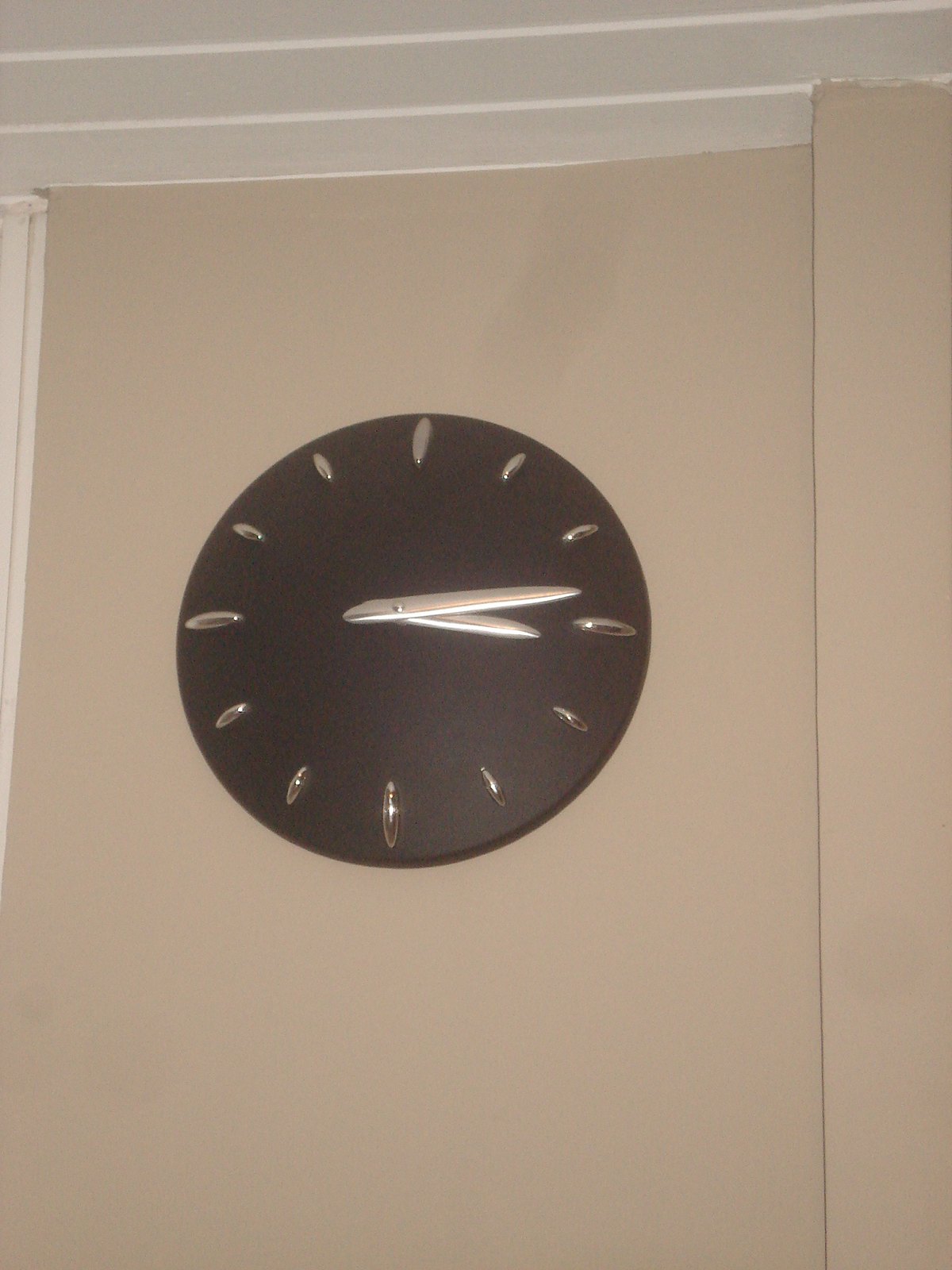A formerly white wall forms the backdrop in the photograph, with a distinct extension on the right-hand side that leads to another pillar. The top portion of this pillar, originally made of white wood, is divided by larger diagonal rectangles, creating a textured visual. Centrally positioned on the wall is a clock featuring silver, pill-shaped markers in place of traditional numerals. There are 12 of these markers, corresponding to the hours on the clock face. The minute hand is positioned between the second and third markers, while the hour hand is slightly past the third marker. Both hands are connected at the center by a small silver dot, completing the minimalist yet striking design.